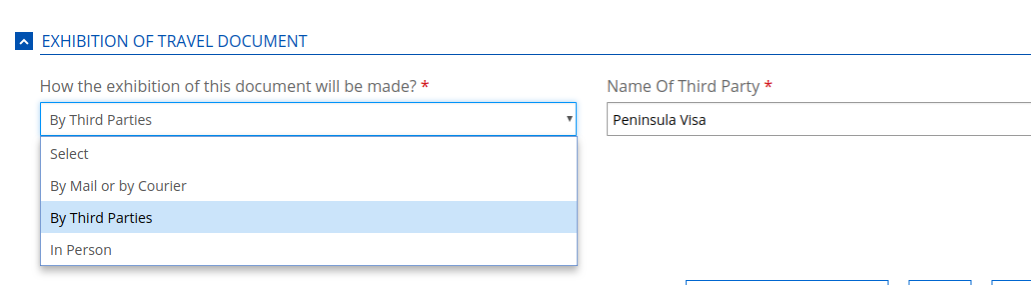**Caption:**

This detailed screenshot captures a section of a website titled "Exhibition of Travel Document," with the title text displayed in blue and accompanied by a small upward arrow icon to the left. Beneath the title, a horizontal blue line visually separates the heading from the content below. The section poses the question, "How will the exhibition of this document be made?" accompanied by a red asterisk indicating that a response is mandatory. 

There is a drop-down menu below the question, offering three options for selection: "By mail or courier," "By third parties," and "In person." The cursor is currently hovering over the option "By third parties." To the right of this drop-down, another mandatory drop-down menu is labeled "Name of third party," also marked with a red asterisk. The currently selected option in this menu is "Peninsula Visa."

Further down, the image shows partial, light blue outlines of buttons, yet the complete content of these buttons is not visible, indicating the screen capture cuts off at this point.